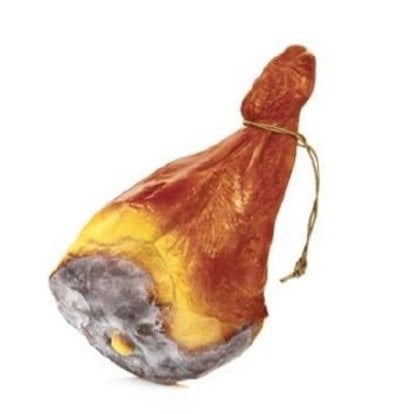The image features a large meat leg, reminiscent of a ham or roasted turkey leg, sitting on its broader base with the bone protruding upwards. The meat is characterized by a dark brown, roasted exterior with a rough, marbled texture, indicating it may be decaying or covered in mold, particularly on the cut surface. The exterior skin transitions from a lighter yellow shade nearer the top to a darker brown further down, ending in a bulbous, knobby end. A string is tied around the narrow upper part of the bone, from which the leg hangs. The bone is also visible at the bottom, protruding slightly and displaying a whitish-gray color, suggesting decomposition or mold. There is no visible background or surface beneath the meat leg.